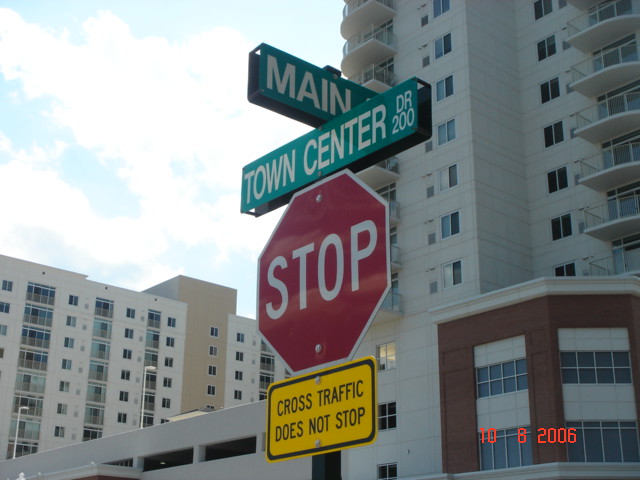The image captures a pole on a street with multiple signs stacked on top of each other. At the top of the pole, there's a green street sign with white text that reads "Main." Directly below it is another green street sign positioned at a 90-degree angle, reading "Town Center Dr 200." Following these is a red stop sign with a white border, displaying the word "Stop" in large white letters. Beneath the stop sign is a yellow and black sign that states "Cross Traffic Does Not Stop." In the background, several buildings appear, resembling either condominiums or apartment complexes, adorned in shades of cream, light brown, and dark brown. One of the buildings, which is closer to the camera and more prominent in the image, features balconies and possibly a parking garage at its base, with brown trim accentuating its structure. The scene is bright, captured on a clear day with a blue sky and some white clouds. In the bottom right corner of the photo, an orange time stamp reads "10-8-2006."